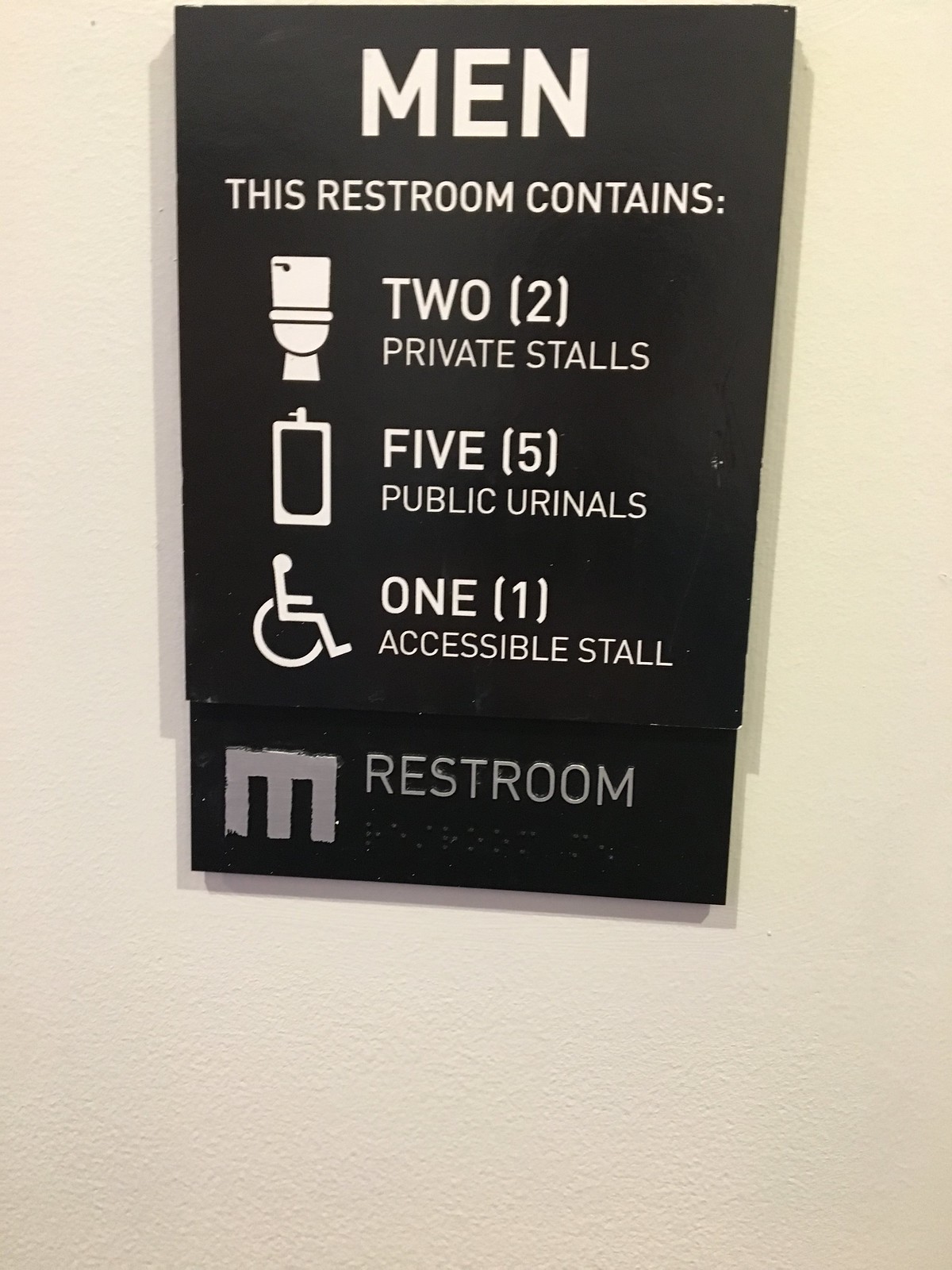This photograph captures a sign mounted on a light-colored wall, which could be described as yellowish-cream or an off-white hue, possibly even light orchid. The sign itself is a deep green or black, possibly with a deep grayish tint, and features white lettering that reads "MEN" in capital letters at the top. The sign details the layout of the men's restroom: it mentions "This restroom contains" followed by illustrations and white text indicating there are two private stalls, five public urinals, and one accessible stall with a wheelchair symbol. At the bottom of the sign, there's a gray capital "M" next to the word "RESTROOM." The sign appears to be somewhat thick, as evidenced by the shadow it casts on the wall behind it.